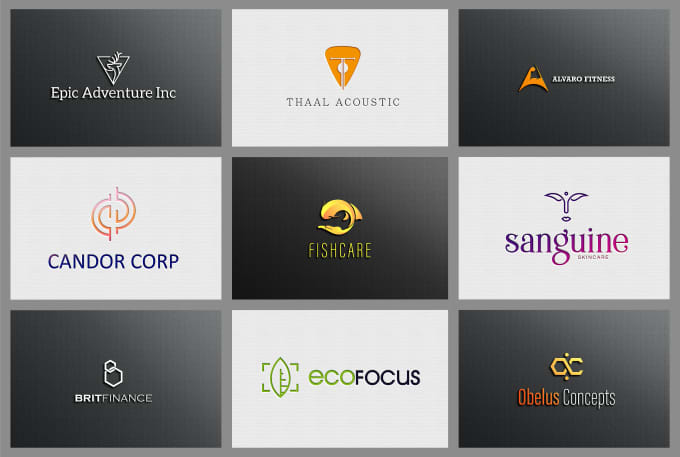This is a detailed image of a chart comprising nine rectangular advertisements arranged in a three-by-three grid, all enclosed by a thick gray border. Each panel is separated by gray lines that match the border. The panels display various vibrant logos and texts, primarily using the colors orange, pink, purple, dark blue, green, and white. The backgrounds alternate between a gray gradient and textured off-white.

Starting from the top left, the first panel features a logo with the text "Epic Adventure Inc." in light gray letters. To the right is a panel with an orange logo that reads "Thal Acoustic" in gray letters, followed by another orange logo that says "Alvaro Fitness" in white letters. 

The middle row begins with "Kandor Corp." on the left, followed by "Fish Care" in the center, and "Sanguine Skin Care" on the right. 

The bottom row includes "Brit Finance" on the left, "Eco Focus" in the center, and "Obelisk Concepts" on the right, which is depicted in orange text. Each advertisement features a unique font and design, highlighting distinctive logos and colors, emphasizing the diverse nature of the represented businesses.